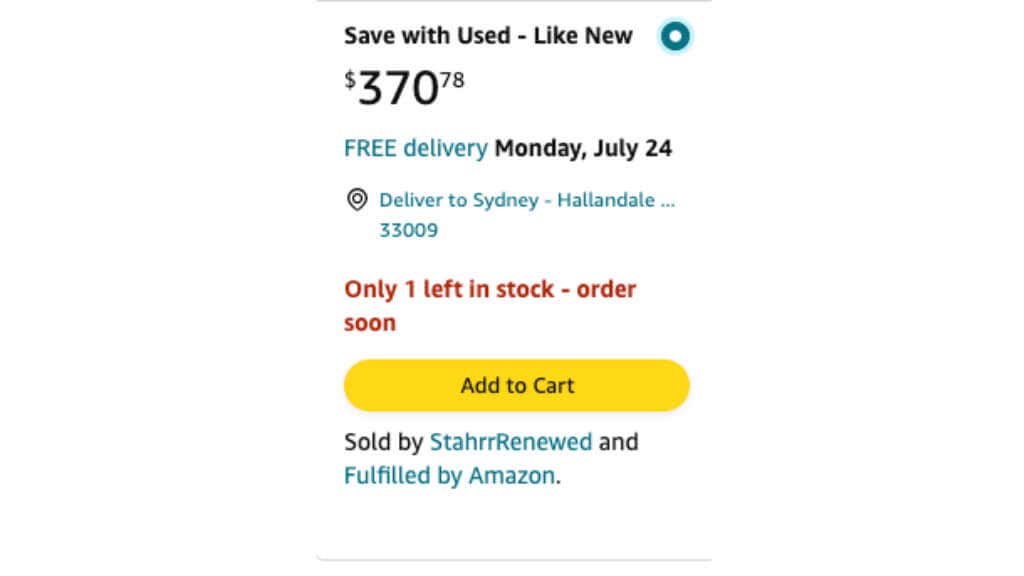The image begins with a light gray line at both the top and bottom. Between these lines, at the top in bold black font, the text reads: "Save with Used-Like New". Adjacent to this, there is a thin turquoise outlined circle that surrounds a darker green-blue circle, which in turn encases a white circle. Inside the white circle, the numbers "370.78" are displayed in black font.

Beneath this, the text "FREE DELIVERY" appears in turquoise, with "FREE" in all caps. To the right of this, in black font, it is stated: "Monday, July 24". Following this is a small black icon.

Below, in turquoise-green text, is the delivery information: "Deliver to Sydney-Hallandale 33009". Continuing downwards, in slightly larger orange font, the message reads: "Only one left in stock - order soon".

At the bottom part of the image, there is a horizontally stretched oval-shaped rectangle with the text "Add to Cart" in black font. Below this, "Sold by" is written in black font, followed by the turquoise text "STAHRENWED" (with "S" in "STAHRENWED" and "R" as capitals). Finally, it is noted in the same turquoise font that the item is "Fulfilled by Amazon".